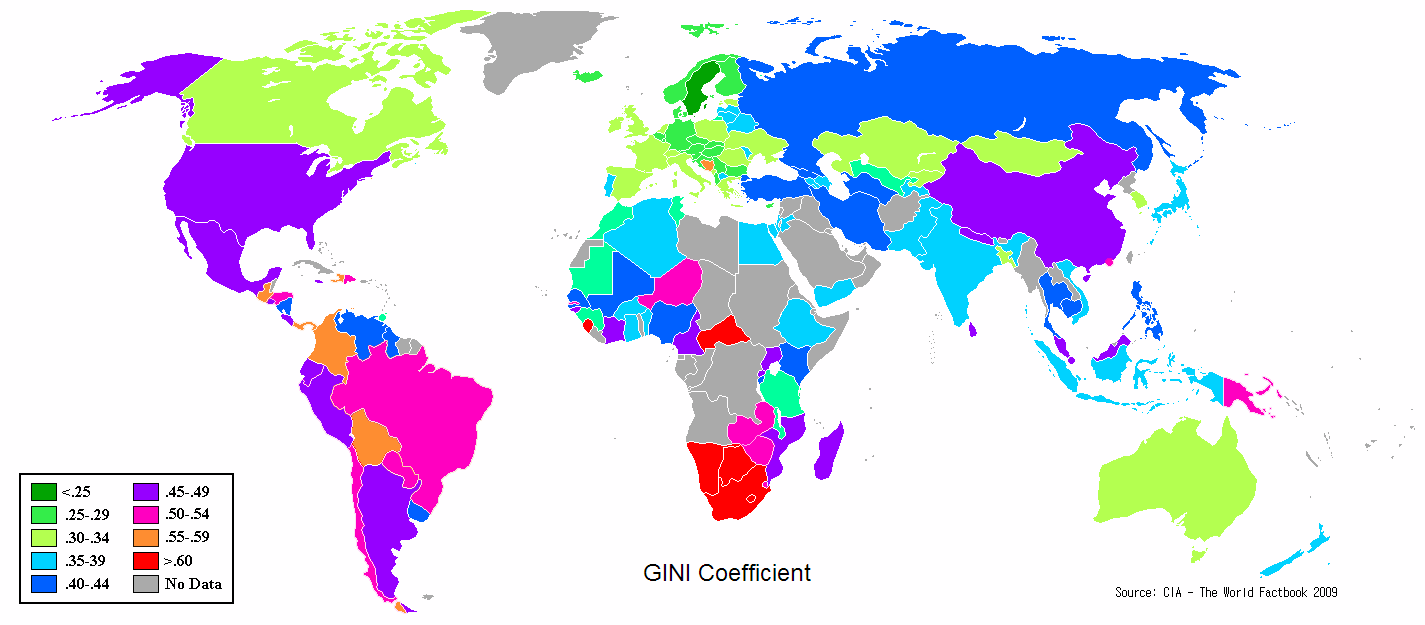This vibrant, detailed map of the world showcases each country in bold, distinct colors. North America is positioned in the top left, with Canada's lime green hue and the United States in dark purple. South America stretches from the middle left, while Africa is prominently centered. Europe and Asia are situated in the top right, with China depicted in purple. Australia, in lime green, is found in the bottom right. The map flattens the globe onto a single plane, creating an eye-catching display of geographical boundaries.

Each country is highlighted in a unique color, such as lime green, purple, pink, red, and blue, providing a striking visual differentiation. However, despite the presence of a color-coded legend featuring numerical values, it lacks specific explanations. At the bottom of the map, the term "Gini Coefficient" is prominently displayed, though its precise meaning and relevance to the numerical values remain unclear. This map offers a visually vivid, albeit somewhat enigmatic, representation of the world's countries.